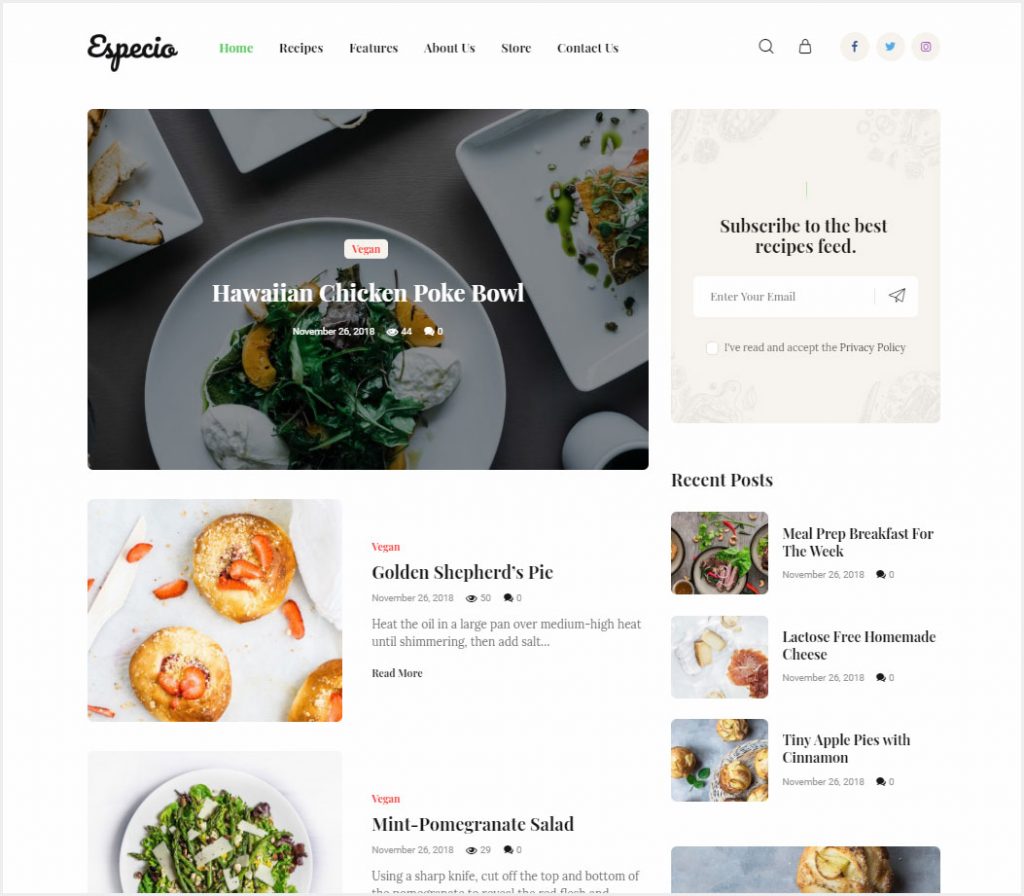The image features a website interface. In the upper left corner, there is bold cursive text displaying the word "Aspecio." To the right of this, a navigation bar includes the following tabs: Home, Recipes, Features, About Us, More, and Contact Us. In the upper right corner, there are icons for a magnifying glass (search), a shopping bag, Facebook, and Twitter.

Below this header is a large, colorful photograph. The image prominently displays a round plate positioned at the bottom of the photo. The plate contains a vibrant salad with sliced oranges and some type of meat. Overlaying this image, the text reads "Hawaiian Chicken Poke Bowl" with a date of November 26, 2018. Above the word "Chicken," there is a small red box with the text "Vegan" inside.

In the lower right corner of the image, there is a section labeled "Recent Posts." The posts listed include "Meal Prep Breakfast for the Week" dated November 26, 2018, and "Lactose-Free Homemade Cheese" also dated November 26, 2018.